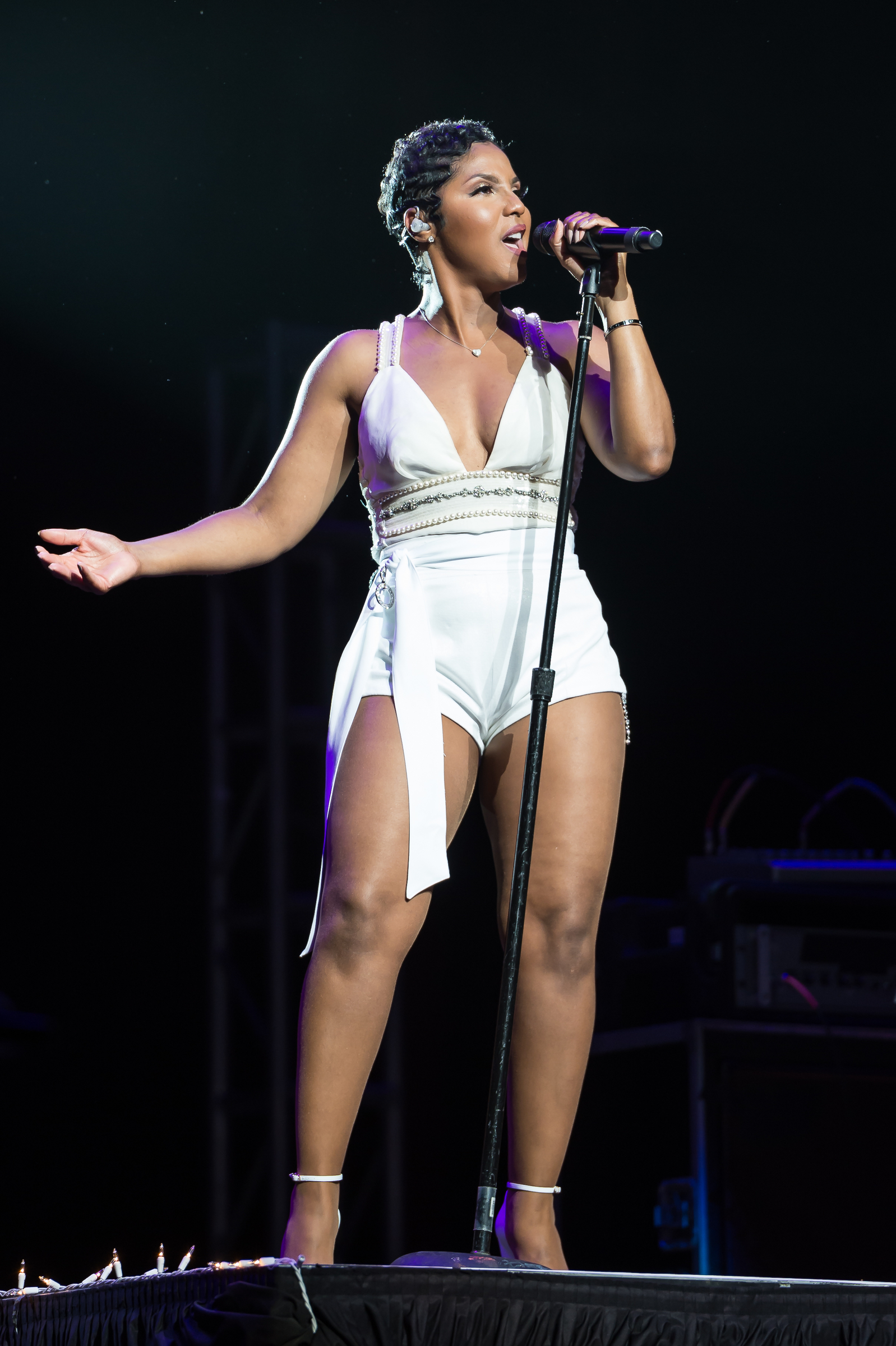In the photograph, a young African-American woman, possibly an iconic singer like Aretha Franklin, is captured mid-performance. She stands alone on a darkened stage, holding a black microphone stand close to her mouth with her left hand, while her right hand extends expressively to her side. She is dressed in a striking white jumpsuit that is short and sleeveless, showcasing her medium-toned skin and a bit of cleavage. The outfit features a white belt tied at her right knee, complemented by white heels and silver, diamond-encrusted accents, including an ear monitor. Her short, dark curly hair frames her face subtly made up, adding to her powerful stage presence. The background reveals minimal stage setup with a black curtain and subtle decorative lights, along with visible scaffolding and some backstage equipment, indicating a sparse setting. She appears deeply immersed in her performance, passionately engaging with the crowd.